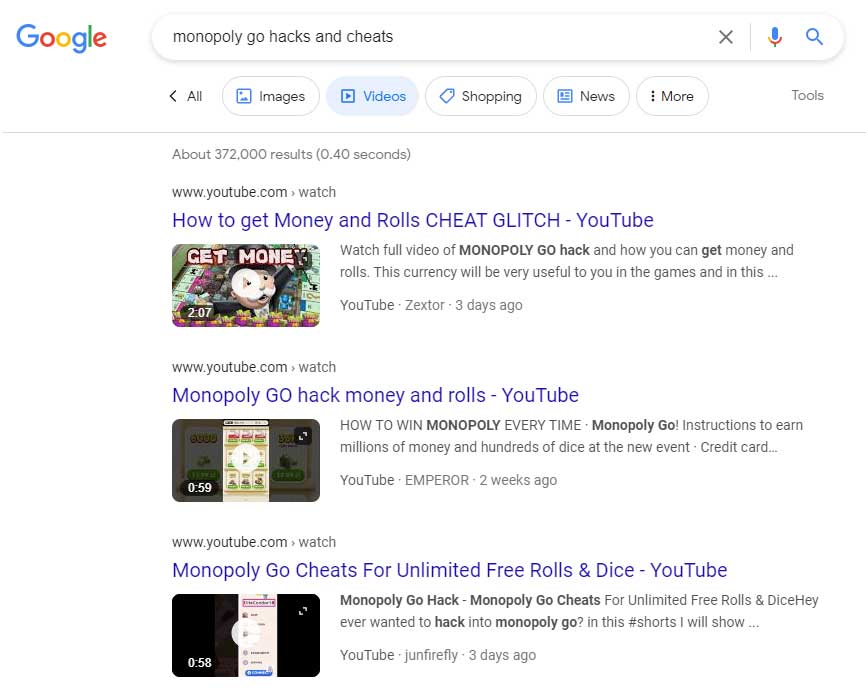The image depicts a Google search results page. At the top left corner, the classic colorful Google logo is visible. To its right is the search bar, where a user has typed "monopoly go hacks and cheats." The search bar features a small "X" icon to clear the text and a microphone icon for voice search. 

Below the search bar is a row of navigational buttons, including "All," "Images," "Videos," "Shopping," "News," "More," and "Tools." The "Videos" tab is selected, indicating that the user is specifically looking for video content on the topic.

The search results indicate that approximately 372,000 results have been found in 0.40 seconds, displayed in a light gray font. The top three video results are listed beneath this information. 

The first video title reads, "How to Get Money in Rolls: Cheat Glitch," and directs users to YouTube to watch the full video. The second video is titled, "Monopoly Go Hack: Money in Rolls," also available on YouTube. The third video, "Monopoly Go Cheats for Unlimited Free Rolls and Dice," is similarly hosted on YouTube.